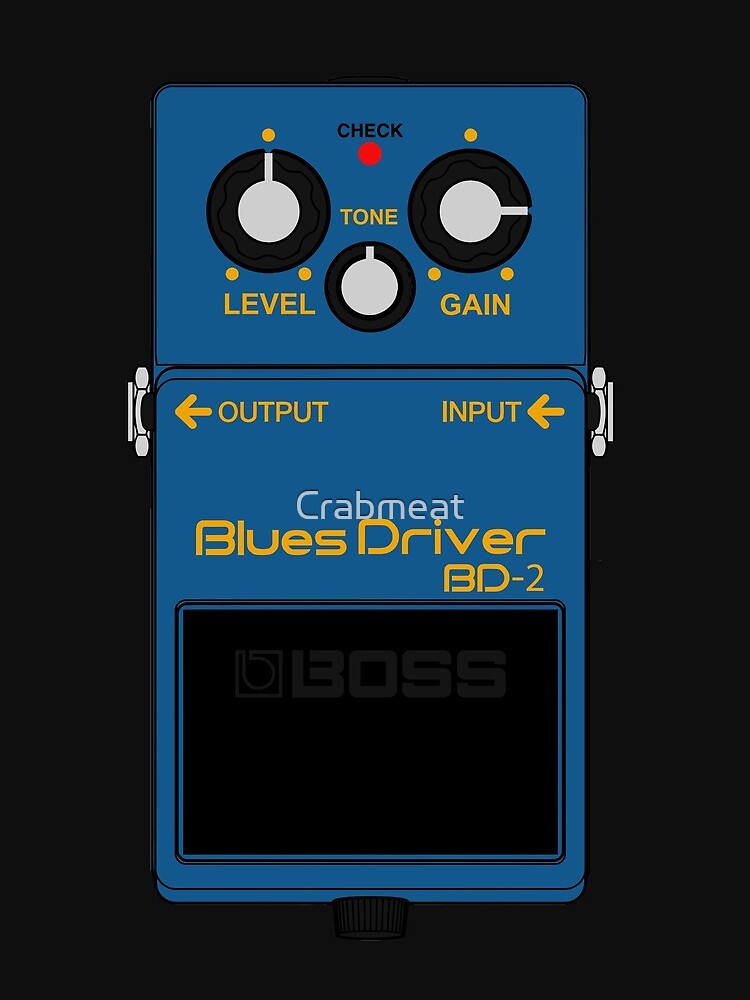In this computer-generated drawing, we see a vertically aligned rectangular device with a detailed design on a solid gray background. The image features a blue, two-sectioned rectangular gadget with a shorter top section and a longer bottom section. 

The top section has three circular knobs. In the center, there’s a small red button labeled "CHECK" in uppercase black letters. Flanking this in larger black circles with white centers, the left knob is marked "LEVEL" and the right knob is labeled "GAIN," both in bright yellow uppercase letters. Below these, a slightly smaller knob in the center reads "TONE."

The lower section of the device showcases the terms "OUTPUT" and "INPUT" with left-facing arrows. The word "CRABMEAT" is prominently displayed in white, followed by "BLUES DRIVER" in yellow and "BD-2" in smaller text underneath. The bottom of this section features a black screen with the name "BOSS" subtly faded in gray lettering. On either side of the device, white fasteners are visible, securing the device components.

This intricately designed piece of equipment appears to be a specialized sound or musical effects pedal, rendered with attention to precise details and labeled functionality.